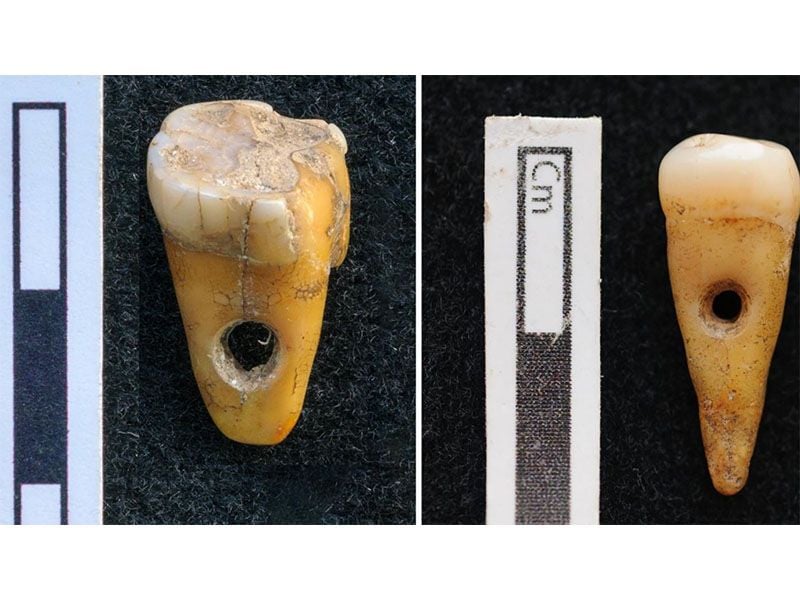The photograph depicts two close-up images of tooth-like objects on a black, felt-like background. Both objects are accompanied by white labels on their left sides, featuring a centimeter scale for size reference. The image on the left shows a yellowed, stained tooth-shaped object with a large, drilled hole through the root area. This tooth appears aged, with brown cracks visible on its smooth, worn surface. The object on the right is triangular and resembles an ice cream cone, complete with a rounded top. It too is yellowed with hairline cracks and has a drilled hole through its center. The labelling indicates scale but lacks descriptive text, emphasizing the comparative size of the objects.